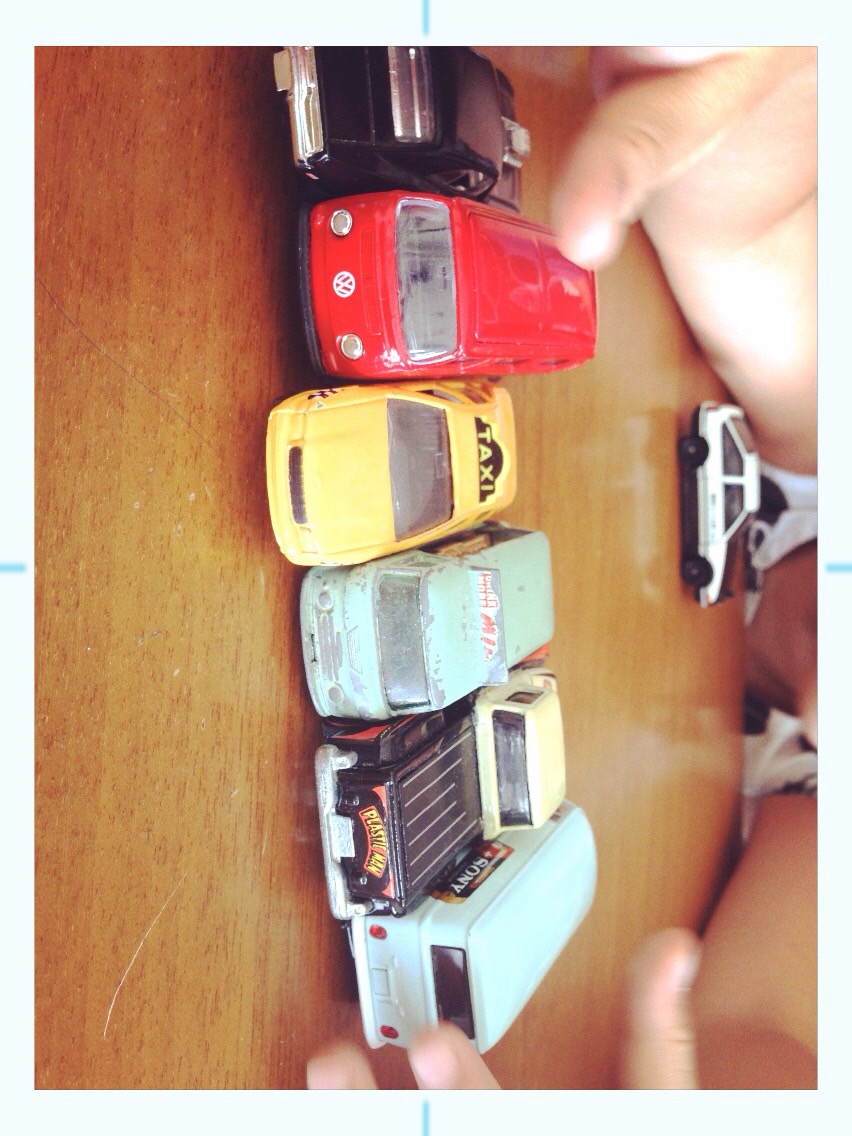In this image, we see a child, identified by their small hands and the bottom of their chin, neck, and a white tank top with black designs. The child is leaning over a shiny, light brown wooden table with some scratch marks, reaching toward an array of toy cars arranged in a line across the surface. Closest to the child's neck in the back of the frame is an old-school, white, and black car with a boxy frame. 

In the front row, from left to right, we have:
1. A black car with a chrome back.
2. A red Volkswagen van with clear glass and two silver headlights.
3. A yellow taxi with the word "TAXI" boldly displayed in yellow over a black background.
4. An old and rusted green van with a faded slogan, likely advertising a beverage.
5. A black and white pickup truck labeled "Plastic Man" on the tailgate, featuring an orange background with yellow letters.
6. Another van, pastel or mint green in color, with a Sony battery sticker on the side.

The child's hands are positioned on either side of the frame, slightly blurred, as they seem to be corraling the toy cars together.